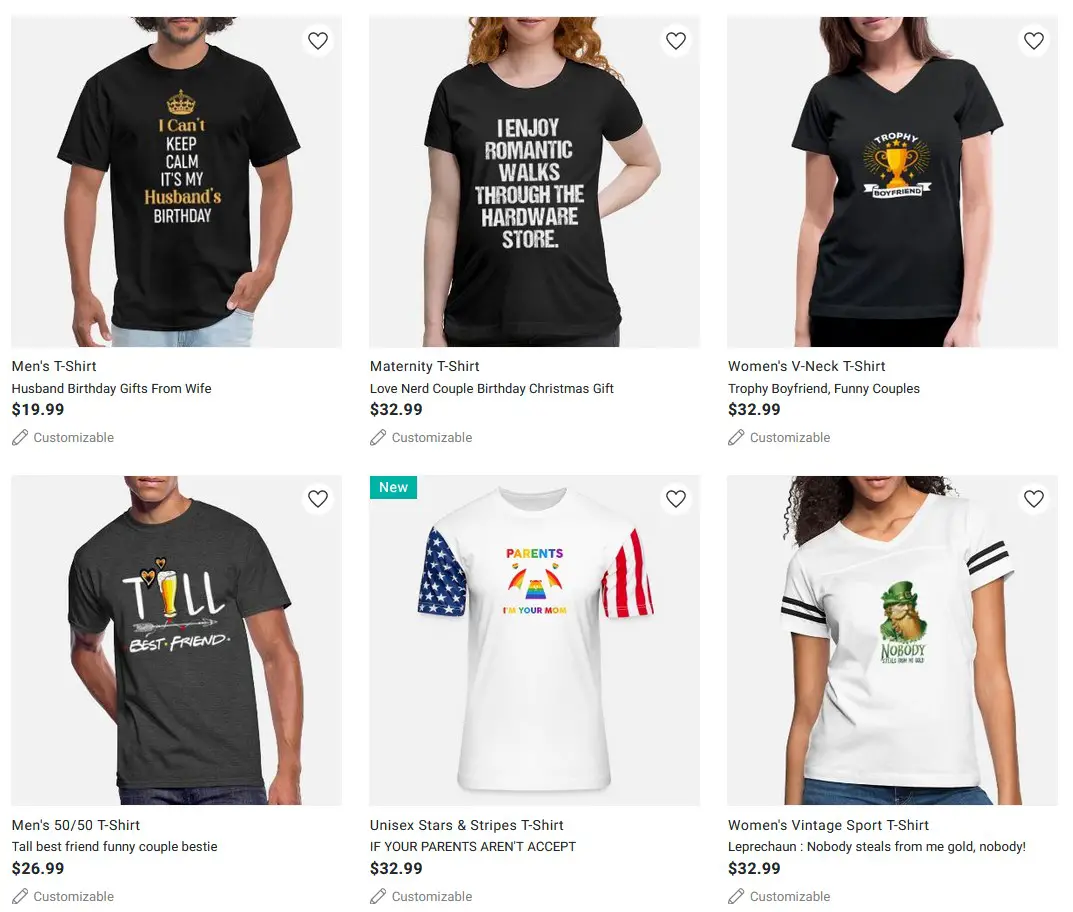This screenshot displays a customizable t-shirt purchasing website featuring six distinct designs. All t-shirts are displayed against a gray background. 

The top row showcases three black t-shirts:
1. The first t-shirt, priced at $19.99, is modeled by a man with curly hair. It features the text "I can't keep calm it's my husband's birthday" in white and gold, with a crown icon above. The words "I can't" and "husband's" are highlighted in gold.
2. The second t-shirt, priced at $32.99, is worn by a woman with curly red hair. The bold white uppercase text reads "I enjoy romantic walks through the hardware store."
3. The third black t-shirt, also priced at $32.99, is worn by a white woman with brown hair. It displays the text "trophy boyfriend" with a gold trophy icon, the rest of the text is in white.

The second row features diverse t-shirts as well:
4. The fourth t-shirt is on a black man and costs $26.99. It reads "Till best friend," with a beer cup icon substituting the letter "i" in "Till."
5. The fifth shirt, priced at $32.99, is white and intended for parents. It says "I'm your mom" in rainbow text, with stars on one sleeve and stripes on the other.
6. The final t-shirt, another white design for $32.99, represents a leprechaun theme and is displayed on a woman with curly hair.

Each t-shirt design is uniquely tailored with different color schemes and textual themes, providing a variety of options for customization.